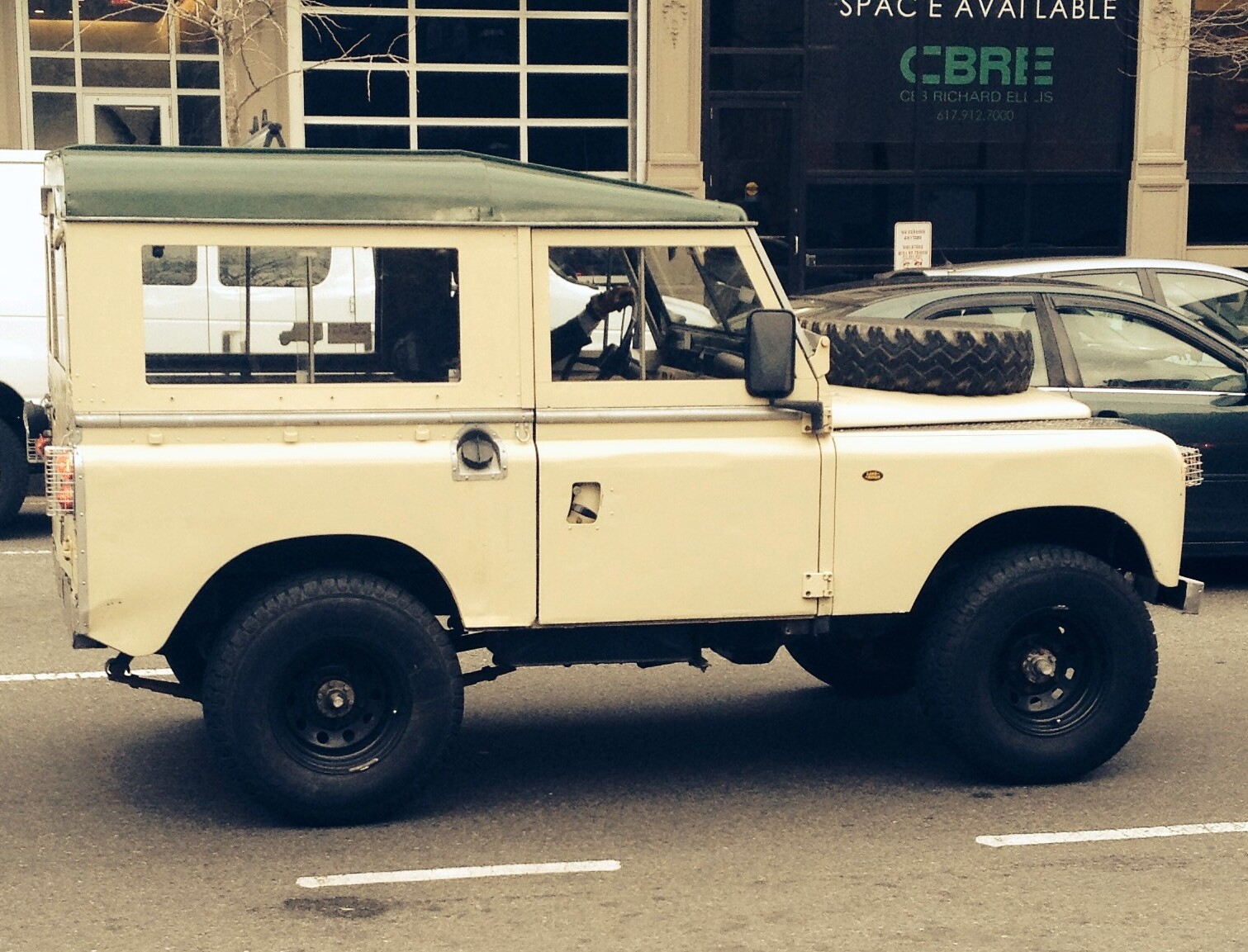The image showcases a bustling urban street scene centered around a vintage tan Jeep with a green roof and a prominent spare tire mounted on its hood. The Jeep, which appears to be stationary amid a traffic jam, features black rims and protective cages around its red lights. A driver is visible inside, with an arm resting through one of the open windows. Flanking the Jeep on the road are a gray hatchback, a black or dark green sedan, and a white van, all halted and facing the same direction. The ground beneath them is a gray road marked by intermittent white lines. The backdrop consists of a tan and black building accented with green, featuring large windows and interspersed pillars. A notable white sign in the building, reading "Space Available, CBRE" in green text, adds a touch of commercial realism to the scene. The overall composition captures the essence of a city street during a moment of pause in traffic.